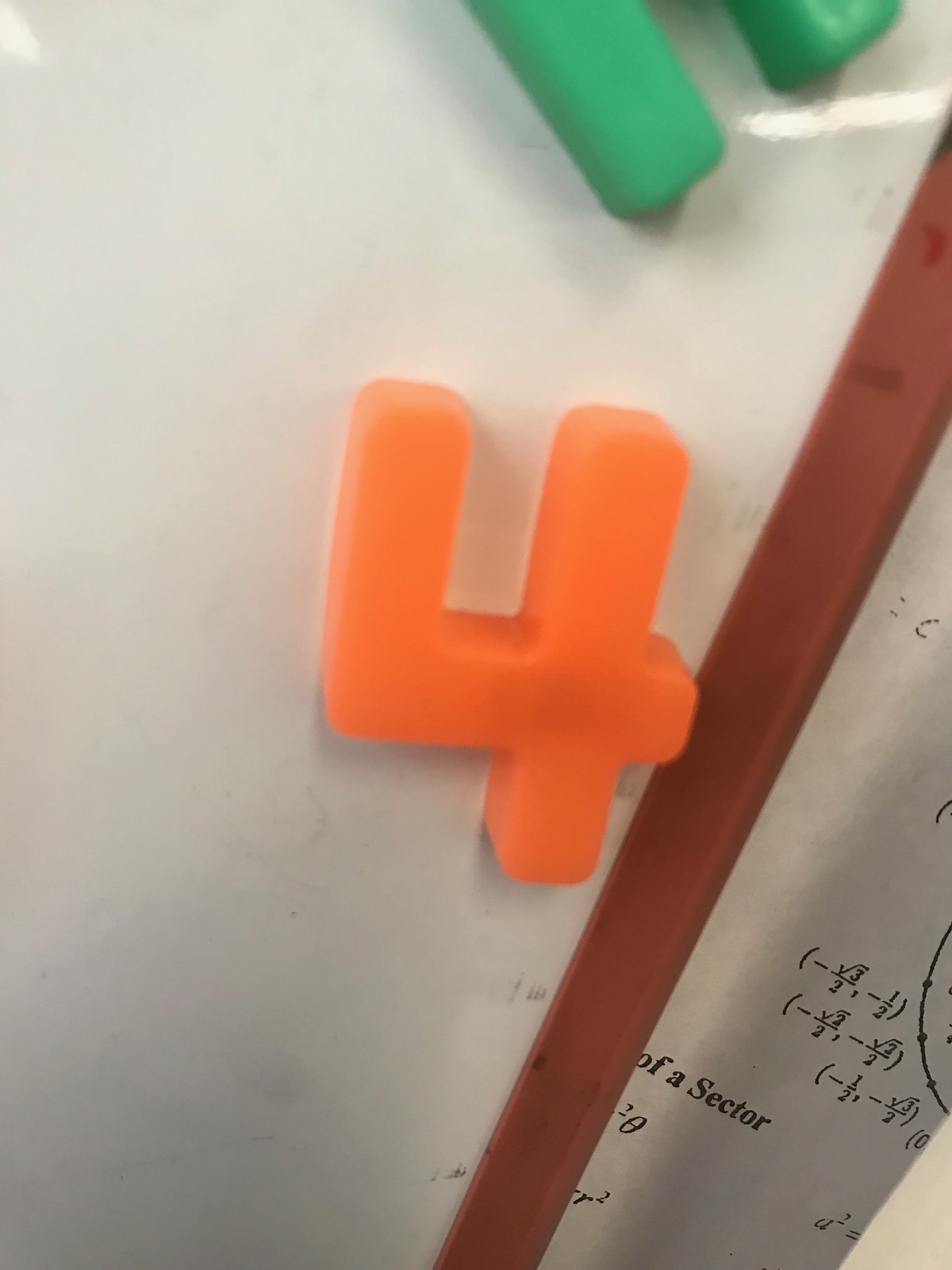The image showcases a close-up of a whiteboard at an angle, featuring an orange, magnetized number four at the center. Above this number four, two small green magnetic objects are visible, partially protruding from the top edge of the image. To the right of these magnets, there is a vertical wooden frame and a section of the whiteboard containing black print text and basic mathematical equations, some enclosed in brackets. The equations and diagrams, which include circles and dots, appear somewhat rudimentary or simplistic in nature.